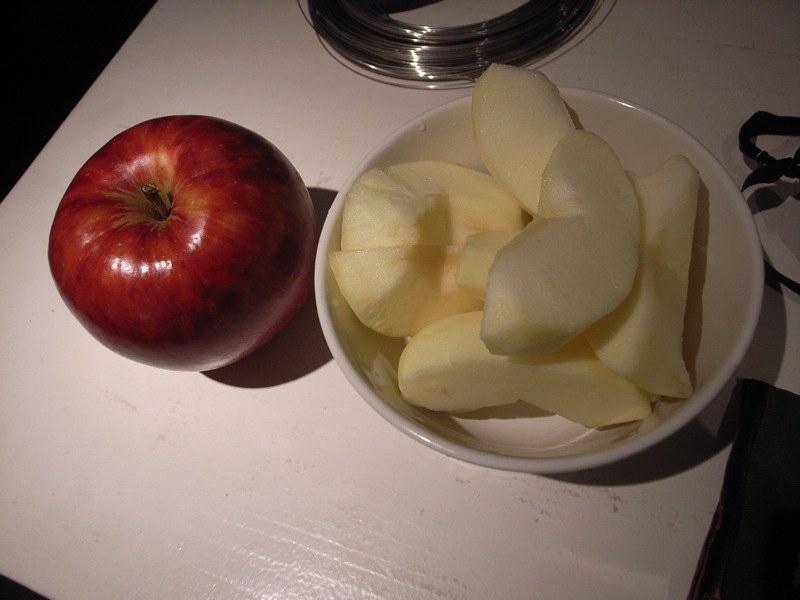In this image, a delectable array of items is displayed on a pristine white table or counter. The table or counter is partially bordered by what appears to be a black placemat, adding contrast to the setting. This placemat can be seen in both the upper left and bottom corners of the picture. On the right side, a section that resembles the strings of an apron adds an interesting texture to the visual.

Prominently featured in the center is a shiny red apple, gleaming under the light. The apple is of an undetermined variety but looks fresh and enticing. To the right of the apple, a white, slightly deep, round bowl is placed. The bowl is filled with neatly cut slices of apple, which have been carefully peeled, revealing their crisp, white interior. This delightful arrangement sits atop what appears to be a silver-colored, wire structure, possibly a trivet, partially visible underneath a layer of clear glass, adding an elegant touch to the presentation.

The composition of these elements—contrast between the black placemat and white table, the vibrant red apple, and the neatly sliced apples in the bowl—creates a visually appealing and harmonious scene, capturing the essence of simplicity and freshness.